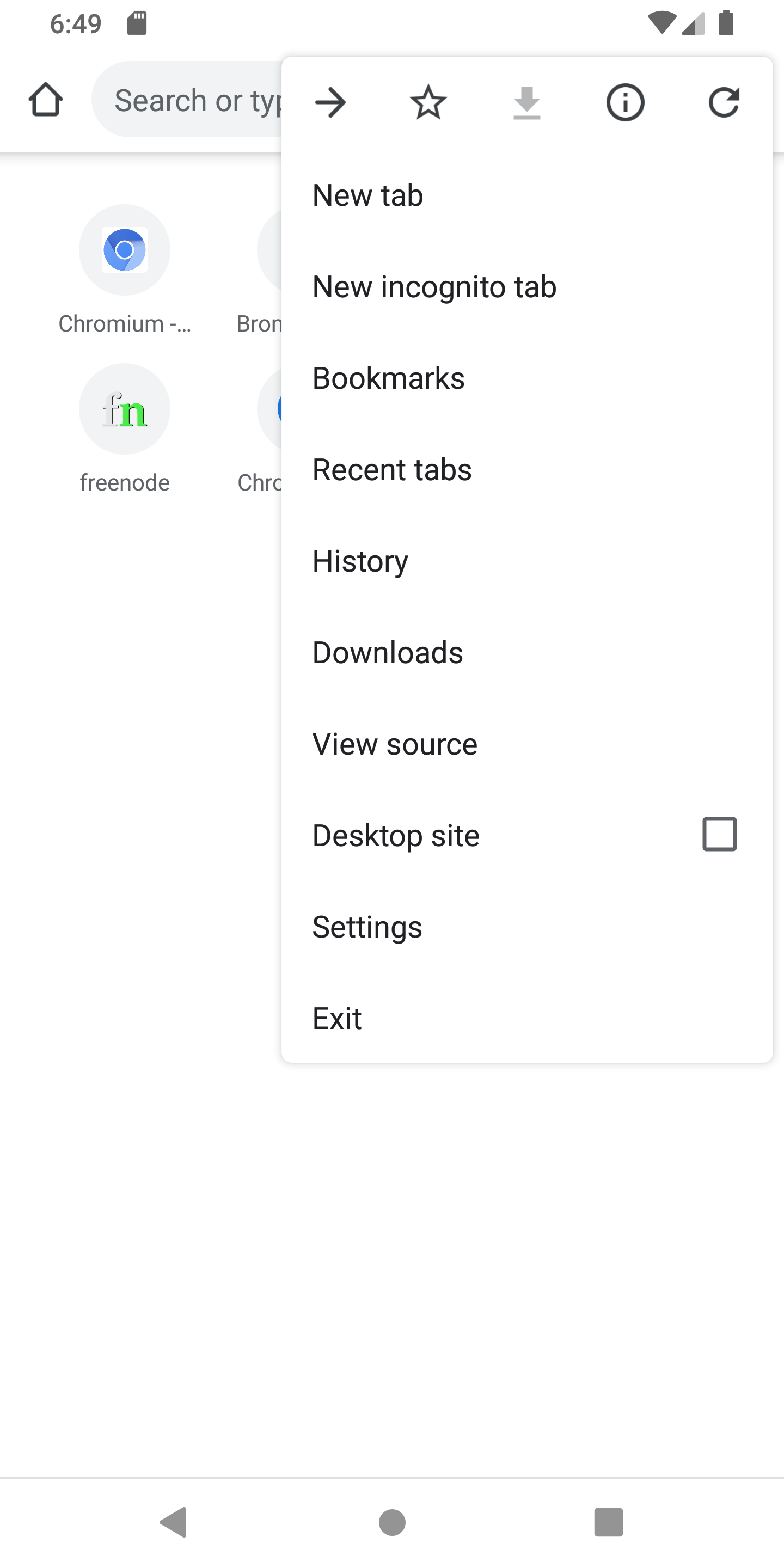In this image, the screen of a smartphone is depicted, showcasing various app icons in the background with a white pop-up box overlaying them. The background reveals several recognizable app icons such as "Chromium," "Free Node," "Chrome," and an incomplete label "BRN." At the top of the screen, a search bar is positioned, accompanied by a home button. The phone’s status bar indicates that the time is 6:49, and the battery is fully charged.

Overlaying the app icons is a white pop-up box featuring several menu options. The top of the pop-up includes a right-pointing arrow, a star, a download arrow, an information icon (a lowercase 'i' inside a circle), and a refresh arrow, all spaced evenly.

The menu options in the pop-up box are listed in the following order: "New Tab," "New Incognito Tab," "Bookmarks," "Recent Tabs," "History," "Downloads," "View Source," "Desktop Site," "Settings," and "Exit." This entire menu is bordered by a thin gray line, forming a rectangle.

At the very bottom of the screen, there is a navigation bar with faint gray lines. The navigation symbols include a triangle on the left, a circle in the center, and a square on the right.